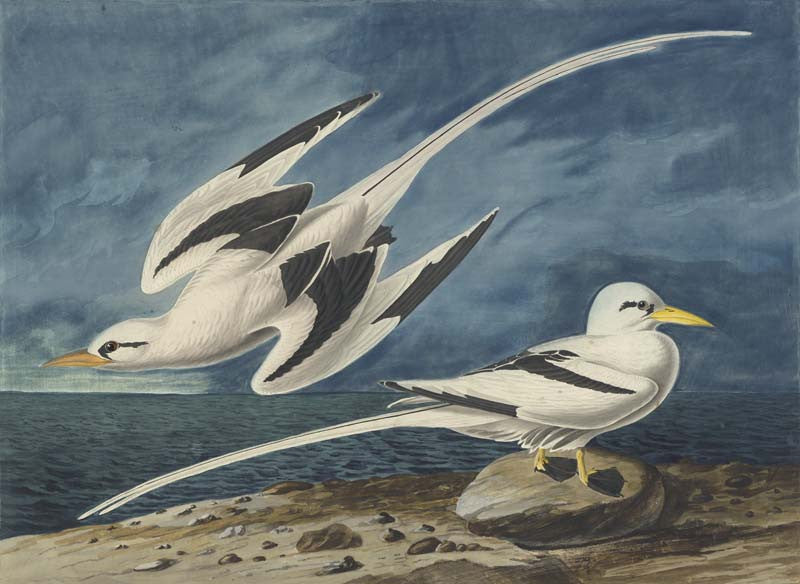This painting, rich in detail and color, depicts a serene coastal scene featuring two distinctive aquatic birds, likely seagulls. Both birds are adorned in striking white plumage with notable black markings: stripes over their eyes and black wingtips, which extend into black stripes across their wings. They have yellow beaks, contrasting with their black webbed feet. One bird is captured mid-flight in the left middle of the painting, its long tail feathers trailing towards the top right corner as it swoops to the left. The second bird stands proudly on a rock amidst a rocky shoreline, its tail extending towards the bottom left corner while it faces right. The varied background features a rippled ocean in shades of medium grayish-blue and dark blue, suggesting cold, deep waters. The sky overhead is a patchwork of medium to dark blue, contributing to the overcast atmosphere. The shoreline, dotted with smaller rocks and some sandy patches, frames the scene, accentuating the natural beauty of the setting against the vibrant colors of the birds and the dynamic ocean backdrop.